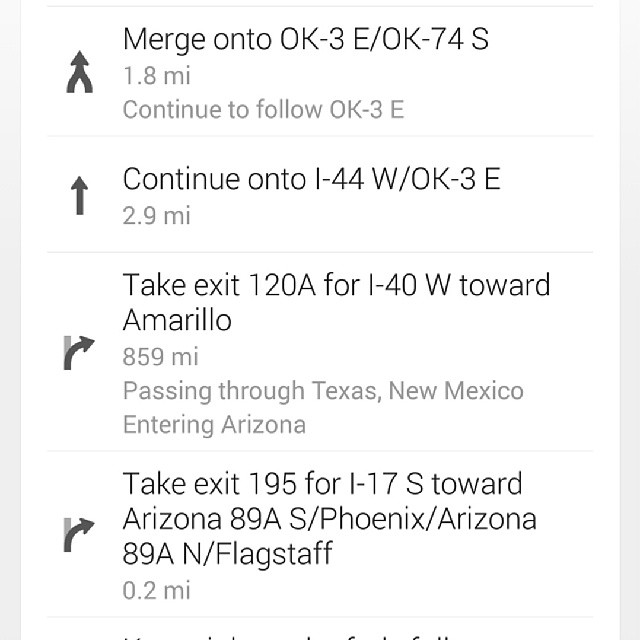### Descriptive Caption for a Vintage Travel Direction Image

The image is a vintage, aged-looking directional chart providing detailed driving instructions from Oklahoma to Arizona. The instructions begin at the top, indicating a merge onto OK-3 / OK-74 South, followed by a continuation onto I-44 West and OK-3E as travelers head towards Amarillo. The route carries on, passing through Texas and New Mexico before entering Arizona. The journey's goal is to take exit 195 for I-17 South towards Arizona 89A, with options to continue South towards Phoenix or North to Flagstaff. The chart is rendered in black font on a white background, with arrows pointing upward, suggesting a direction from Oklahoma to Arizona. If read in reverse, it provides directions from Arizona to Oklahoma. This vintage directional map is both a functional guide and a nostalgic piece of travel memorabilia.